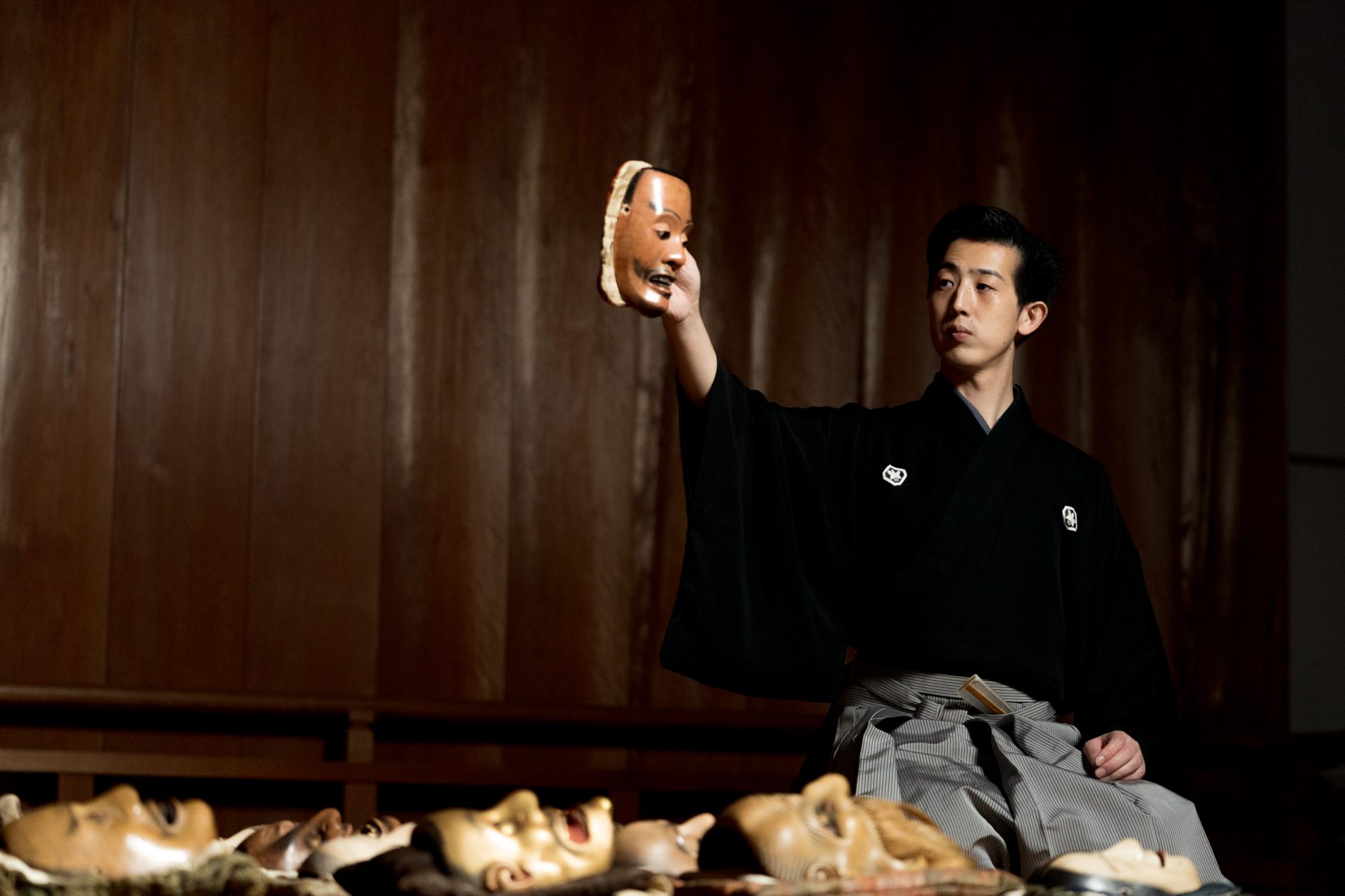This indoor photograph captures an Asian man, likely Japanese or Chinese, sitting on the floor in a kneeling position. He has dark hair and wears a black robe on his upper body adorned with white emblems, which are not fully legible, and light gray pants. A gold loop is visible on his belt. In his right hand, he holds a brown wooden mask with some white detailing. To his left on the floor, a collection of various masks is spread out, displaying diverse expressions and characteristics, such as one with black hair, one with no hair, and another with its mouth open. The setting features a wooden wall of brownish-red hue behind him, adding a warm tone to the scene. The overall lighting of the image is dark, enhancing the contrasting colors of black, white, gray, beige, and brown throughout the composition.